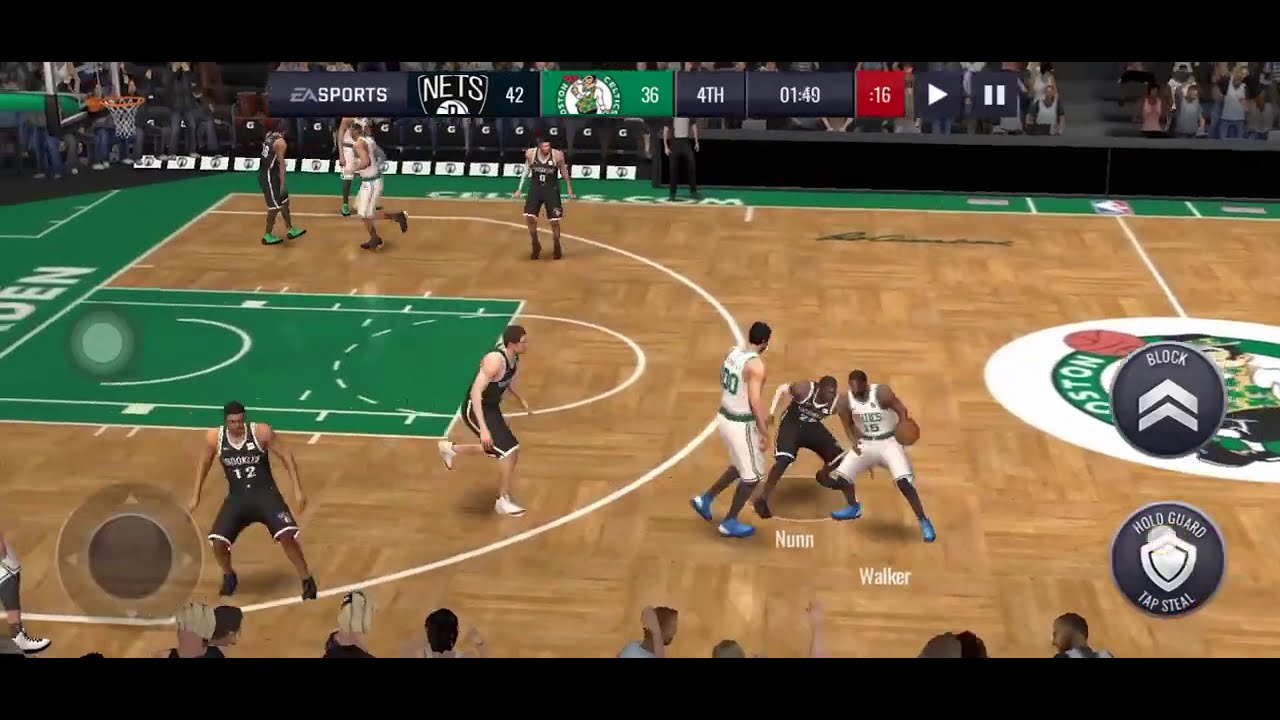This image is a detailed screenshot from an NBA video game. The scene displays a high-intensity basketball game between the Boston Celtics and the Brooklyn Nets, highlighting the action during the fourth quarter with 1:49 remaining on the clock. The Celtics, dressed in white and green jerseys, are competing against the Nets, who are wearing black and white. Dominant in the center, three players are engaged—one dribbling the ball while a defender from the Nets attempts to steal it, and another Celtics player setting a screen. Notably, the players' last names "Nun" and "Walker" are visible on their jerseys. Surrounding the main trio, about five other players are positioned sporadically, contributing to the game's dynamic. The basketball court features a wooden parquet design with a green perimeter and a Boston Celtics logo at center court. The court is bordered by a green free-throw area, while a red background highlights the shot clock countdown. The interface displays control options such as block, hold guard, and tap steal at the bottom right. Branding elements include an EA Sports banner and the game's score displayed at the top, where the Nets lead with 42 points against the Celtics' 36. The subtle crowd and the green bordered arena further immerse the viewer into the game.